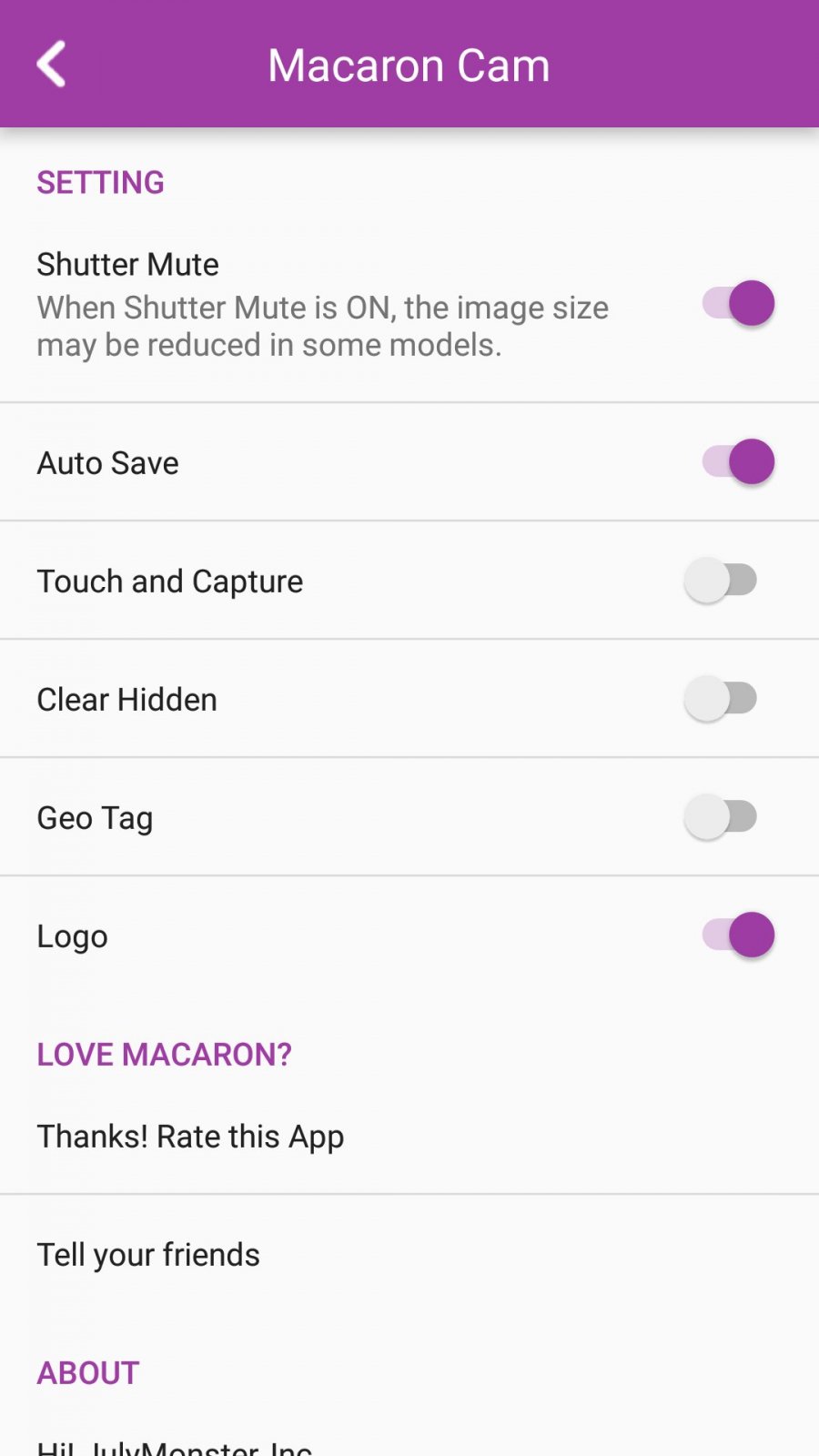This image shows a screenshot of the settings page from the "Macaron Cam" app on a mobile phone. At the top is a purple bar with white text that reads "Macaron Cam," accompanied by a white left-pointing arrow on the left side of the bar. Below the bar, the page header "Setting" is prominently displayed in purple font on a white background.

The settings are listed as follows:

1. **Shutter Mute**
   - Description: "When Shutter Mute is on, the image size may be reduced in some models."
   - Status: The purple toggle switch is turned on.

2. **Auto Save**
   - Status: The purple toggle switch is turned on.

3. **Touch and Capture**
   - Status: The gray toggle switch is turned off.

4. **Clear Hidden**
   - Status: The gray toggle switch is turned off.

5. **Geotag**
   - Status: The gray toggle switch is turned off.

6. **Logo**
   - Status: The purple toggle switch is turned on.

Beneath these settings, a promotional section appears with the text "Love Macaron?" in blue font, and below it, "Thanks! Rate this app!" in black font.

Each setting is divided by a black line for clear separation, and the toggles indicate the current status of each feature. The interface is clean and well-organized, making it easy for users to navigate and adjust their preferences.